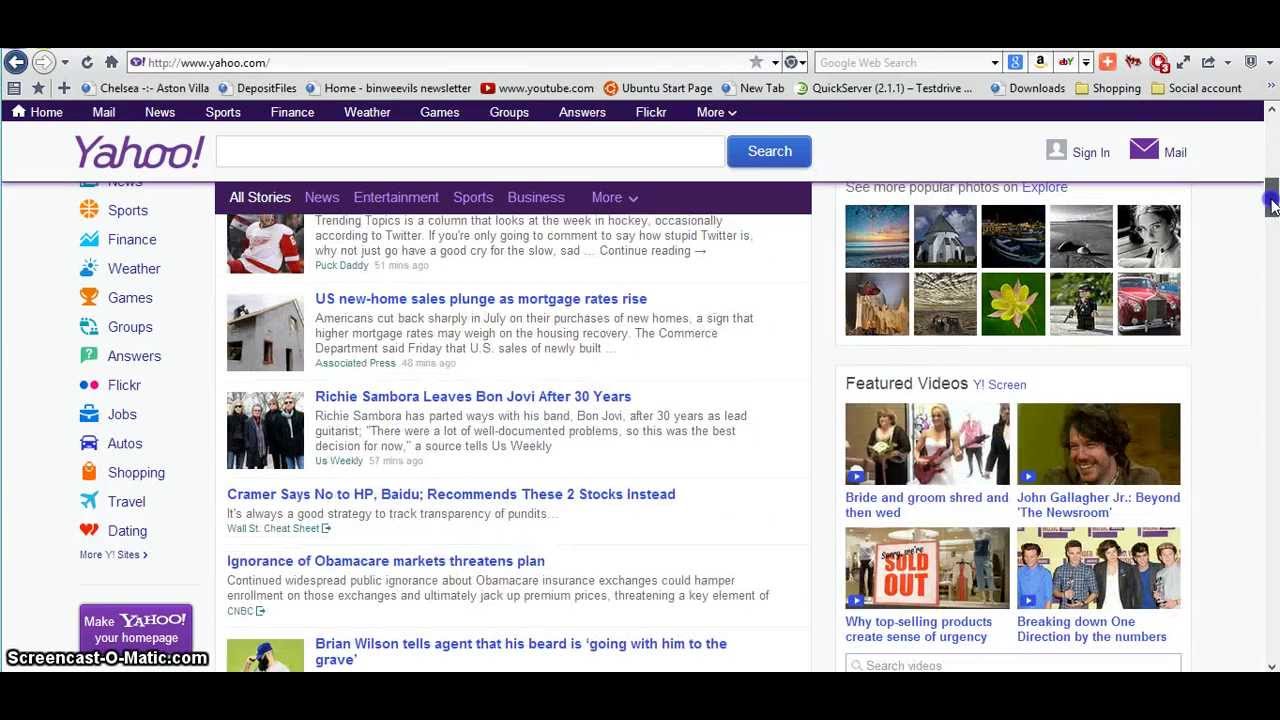The screenshot displays a webpage with black bars at the top and bottom. At the top left, there are left and right arrow icons, followed by the URL "http://www.yahoo.com." The central area of the screen appears to be a search results page or a portal page featuring a variety of links and sections.

In the upper part, there are icons and links for popular websites and services such as Google, Amazon, and eBay. There's a red square present, possibly representing a notification or a featured link. Other names mentioned include Chelsea, Ashton Villa, Deposit Files, Home, Ben Rose, Dizzler, YouTube, Uber, and G-Tag.

On the right side, there is a menu listing options like Quick Server, Test Drive, Download, Shopping, Social Account, Home, Mail, News, Sports, Finance, Weather, Games, Groups, Answers, Flickr, and more.

Below, there is a Yahoo sign-in section with options for accessing Mail. Another column lists categories including Sports, Finance, Weather, Games, Groups, Answers, Flickr, Jobs, Auto Shopping, Travel, and Dating.

The main content area consists of news and information such as:
- U.S. New Home Sales and Mortgage Rates.
- Articles on Riches and Morellis, Bon Jovi, and a quote from Kramer saying "no" to HP.
- Biden's stock recommendations and a critique of Obamacare.
- Market updates and plans.

A featured video section showcases screencasts on medec.com with content about John Gallagher and a segment titled "Beyond the Visual." There is also mention of top-selling products, tenant information, and a breakdown of the band One Direction.